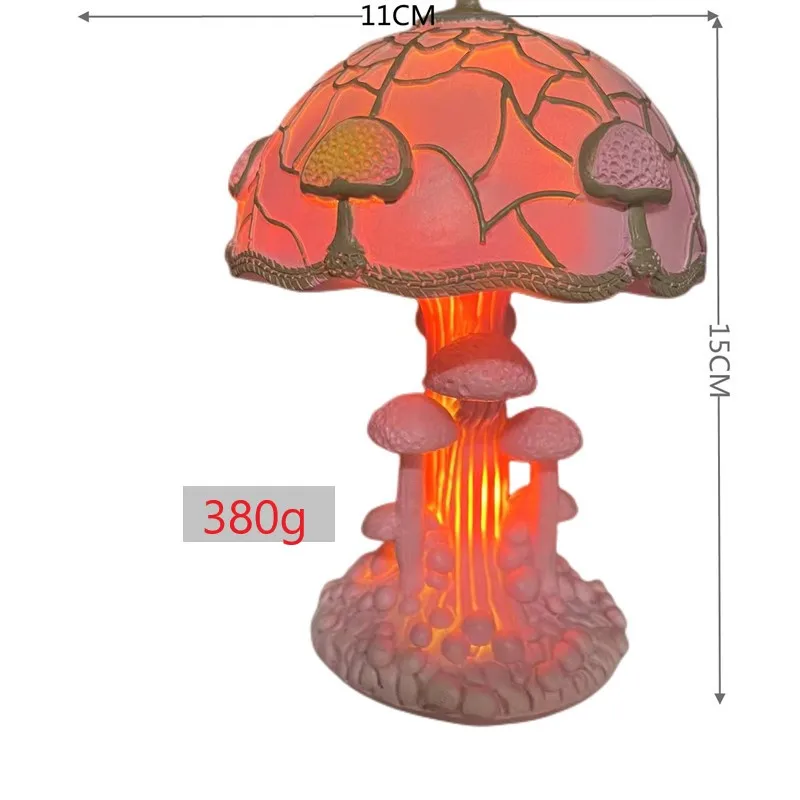The image features a uniquely designed lamp, modeled to resemble a mushroom. The lamp’s stem serves as the light source, illuminating in a glowing orange hue, though the exact color of the stem when unlit is unspecified. Clusters of small mushroom-like protrusions adorn the stem and its base, adding a whimsical touch. The lamp’s top resembles an umbrella and is designed like a mushroom cap, complete with detailed green lines that contrast beautifully with the orange glow when the lamp is turned on. Measurement indicators are present on the right side of the image: the height of the lamp is marked at 15 cm, and its width at 11 cm. Additionally, a gray rectangle on the left side specifies the lamp’s weight as 380 grams, highlighted in red text.